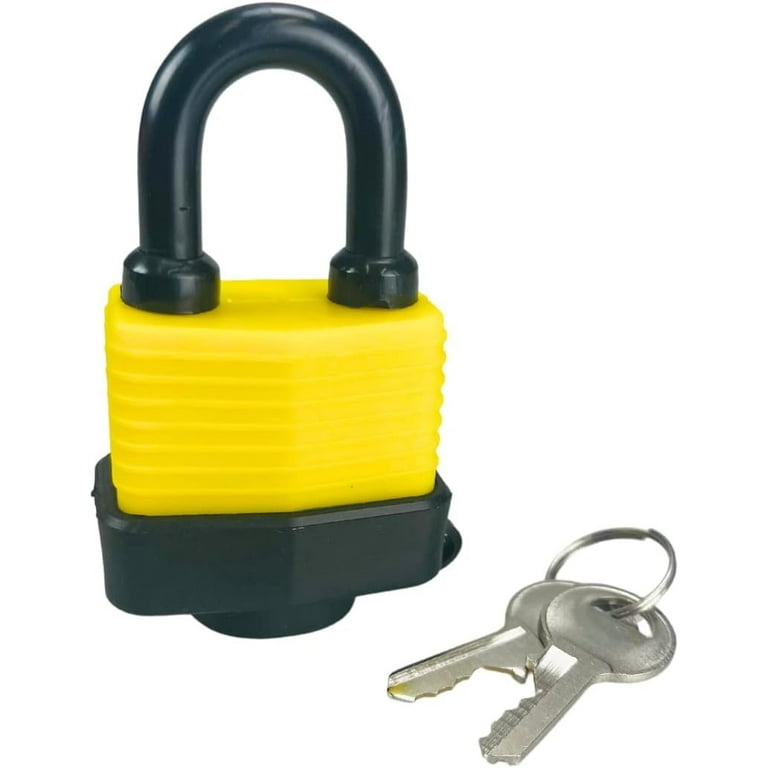The image depicts a brightly lit, close-up view of a padlock situated on a clean, white background. The padlock, positioned on the left-hand side of the image, features a distinct yellow body seamlessly integrated into a protective black base. The lock's shackle, an upside-down U shape, is black and attaches at the top of the yellow body. Adjacent to the lock, two silver keys rest flat on the white surface to the lower right of the padlock. The teeth of these keys face inward towards each other and are held together by a small, circular silver keychain. No text or numbers are visible, and no extraneous objects detract from this clear, focused scene.